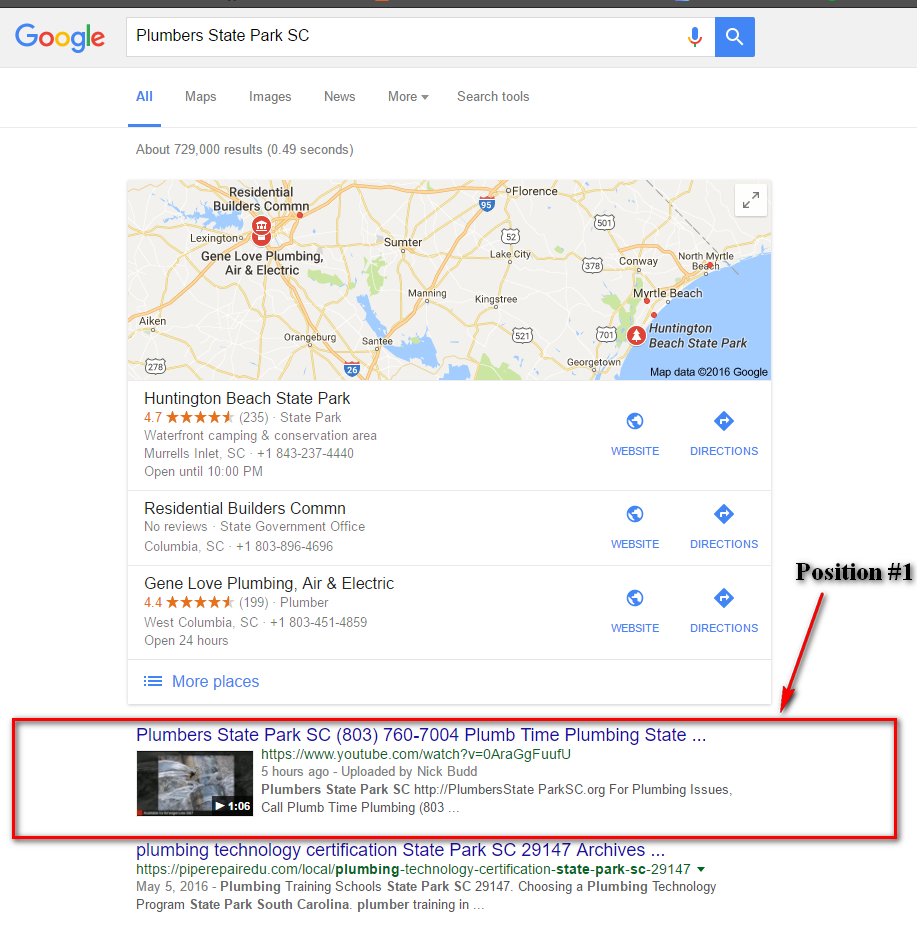This image depicts a Google search results page. The Google logo is prominently featured in the top left corner, with each letter colored differently: the first "G" in blue, the first "O" in red, the second "O" in yellow, the second "G" in blue, the "L" in green, and the "E" in red. The search query "plumber Stakes Park SC" is typed into the search bar, which is flanked by a microphone icon on the right and a search icon.

Below the search bar, there are navigation tabs for different types of results: "All," "Maps," "Images," "News," and "More." The "All" tab is currently highlighted. Directly beneath these tabs, the page indicates there are about 729,000 results available, found in 0.49 seconds.

The first part of the search results features a map and several location listings. For example, "Huntington Beach State Park," rated 4.7 stars, is one of the highlighted places. Additionally, "Gene Love Plumbing and Electric," rated 4.4 stars, is another notable listing. Each of these entries includes options for accessing their website or getting directions.

The embedded map on the right shows various locations mentioned in the search results. Residential Builders Company and Gene Love Plumbing and Electric are pinpointed on the left side of the map, while Huntington Beach State Park is marked closer to the Myrtle Beach area. Below the map, another search result mentions "plumber Stake Park SC 803 760 7004 Plumb Time Plumbing," highlighted with a green square. A red square annotates the first search position where the primary focus of the search results is indicated.